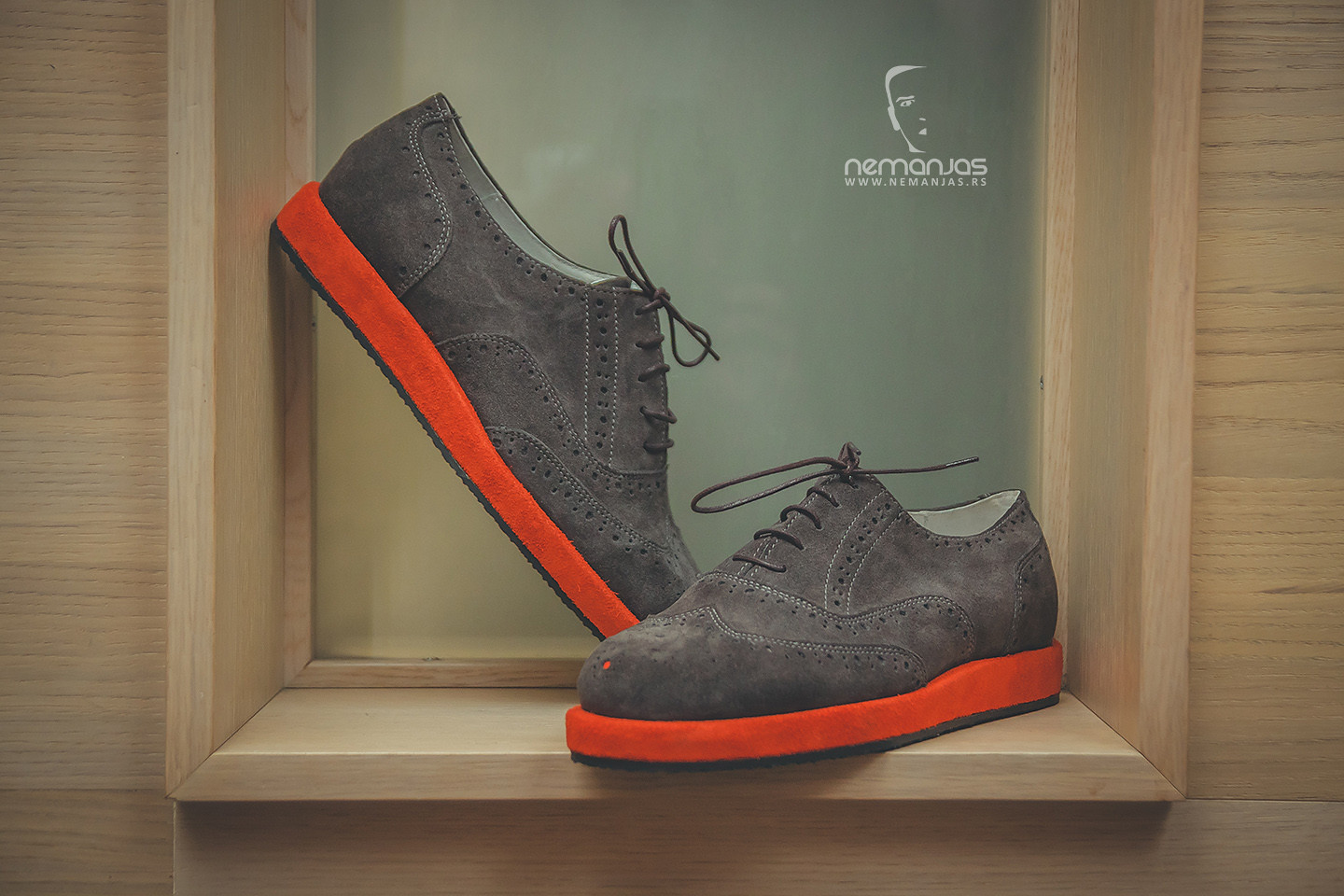This meticulously composed photographic advertisement showcases a luxurious pair of gray suede sneakers, elegantly blending elements of dress and tennis shoes. The setting is indoors, with the shoes artfully displayed within a light tan wooden cubby that features a contrasting light green background. One shoe is positioned flat on the right side of the cubby, while the other is propped up on its heel on the left, creating a visually appealing asymmetry.

The sneakers, which have approximately five well-laced shoelace holes, are bordered along the heel and sole with vibrant red highlights, and they boast bright orange soles, adding a vivid pop of color against their gray suede bodies. The sneakers’ interior appears white, enhancing their sophisticated yet sporty aesthetic.

In the top right-hand corner of the green background, the logo features a sketched face beside the white text "N-E-M-A-N-J-A-S" and the URL "www.nemanjas.rs," capturing the essence of the brand. The landscape orientation and realistic style of this professional product photograph emphasize the elegance and luxury of the sneakers, making them stand out in this carefully crafted advertisement.